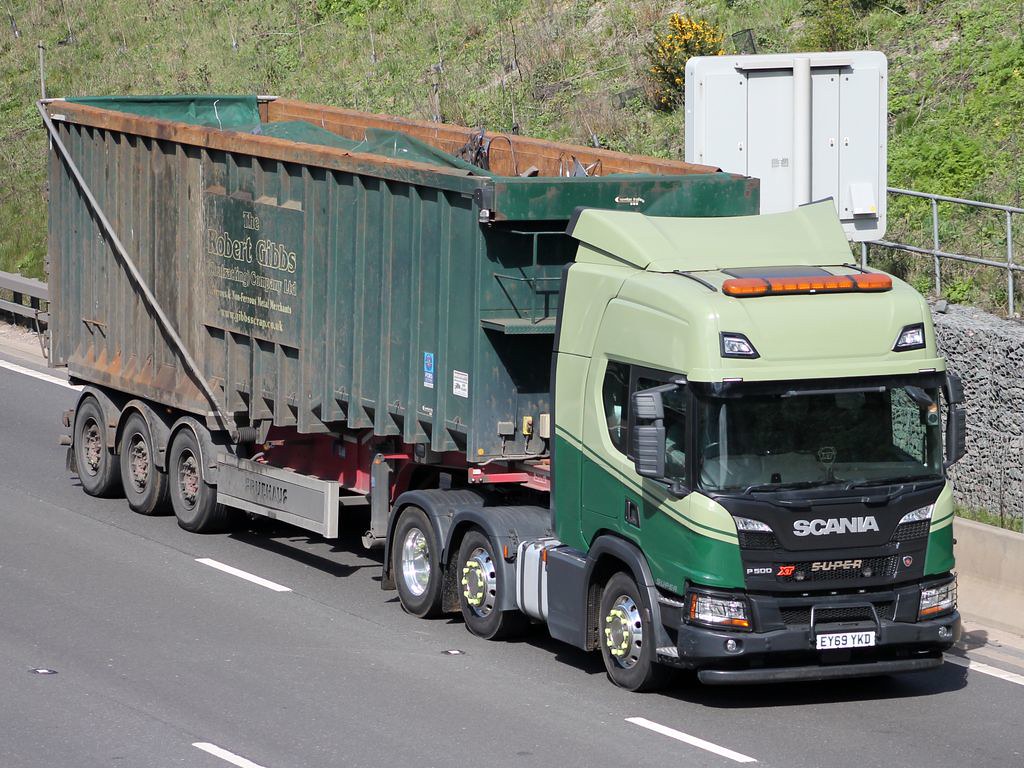The image depicts a European sanitation semi-truck driving down a highway, carrying a green roll-off dumpster that has a green cover, indicating it is full. The truck itself features a two-tone green color scheme, with dark green on the lower part and a lighter green on the top. Notably, the front of the truck bears the silver letters "S-C-A-N-I-A" along with "Super" and "P-500," and the European license plate reads E-Y-6-9-Y-K-D. In the background, there's a lush green hill and a stone wall topped with a metal fence bordering the highway. A white traffic sign is partially visible behind the truck. The dumpster appears slightly dirty or rusted, with hints of red. Orange lights are mounted on the truck, contributing to its utilitarian look.